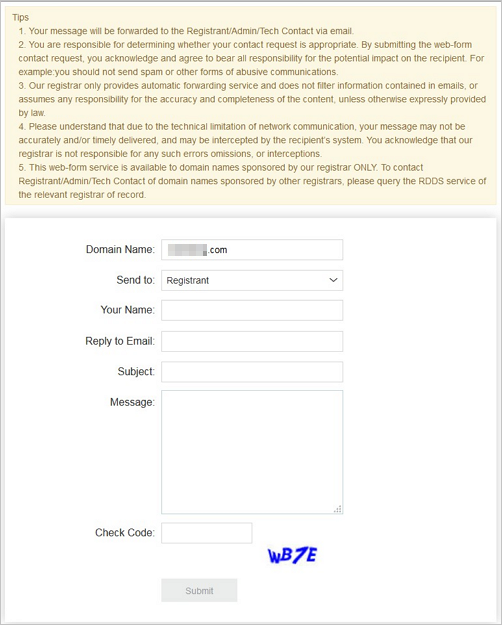**Caption:**

This image is a detailed screenshot of a web-based contact form intended for domain registrants. At the top of the page, a yellow box labeled "Tips" provides crucial information: "Your message may be forwarded to the resident administrative contact via email. It is your responsibility to determine the appropriateness of the contact request before submitting the web form. Misuse, such as sending spam or other unauthorized communications, is prohibited." The section further clarifies that the registrar only provides automatic forwarding services and does not filter the contents of the emails. Due to network communication limitations, messages may not be promptly or accurately delivered and could be intercepted. The service is available exclusively to domain names sponsored by a registrar and not for those under other registers; for such domains, the RDDS service of the relevant registrar should be queried.

Below the information message, the form fields are displayed. The "Domain Name" field shows a blurred domain, "blurredout.com." There are sections to input your name, a "Reply-To" email, the subject of the message, and the message itself. A CAPTCHA code, "WB7E," in blue ensures that submissions are not automated. At the bottom, a "Submit" button is grayed out, awaiting valid input to be activated. 

This contact form serves as a means for web authorities to communicate with domain registrants, while emphasizing the importance of appropriate and legitimate use.